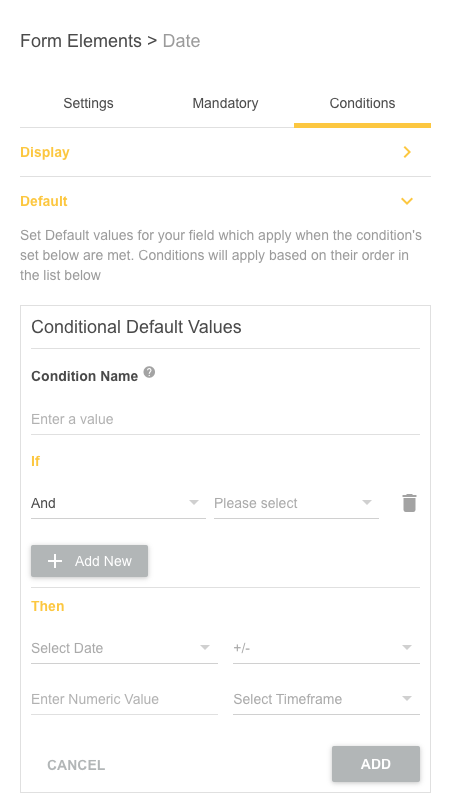Screenshot from a website: 

In the top left corner, black text reads "Form Elements," followed by a triangle icon and the word "Date," all set against a white background. Below this header is a black text navigation menu containing the items: "Settings," "Mandatory," and "Conditions." The current tab, "Conditions," is highlighted with a thick yellow underline. 

Within the "Conditions" tab, a list of various options appears in yellow text. One of these options, labeled "Display," is collapsed and its contents are hidden. The currently selected option is "Default," displayed in yellow text. Beneath the yellow "Default" label, gray text explains: "Set default values for your field which apply when the conditions set below are met. Conditions will apply based on their order in the list below."

Further down, a section outlined in gray is labeled "Conditional Default Values" in black text. This section features several fillable fields labeled "Condition Name," "If," and "Then." At the bottom left of this section, there are two buttons: "Cancel" and "Add Option."